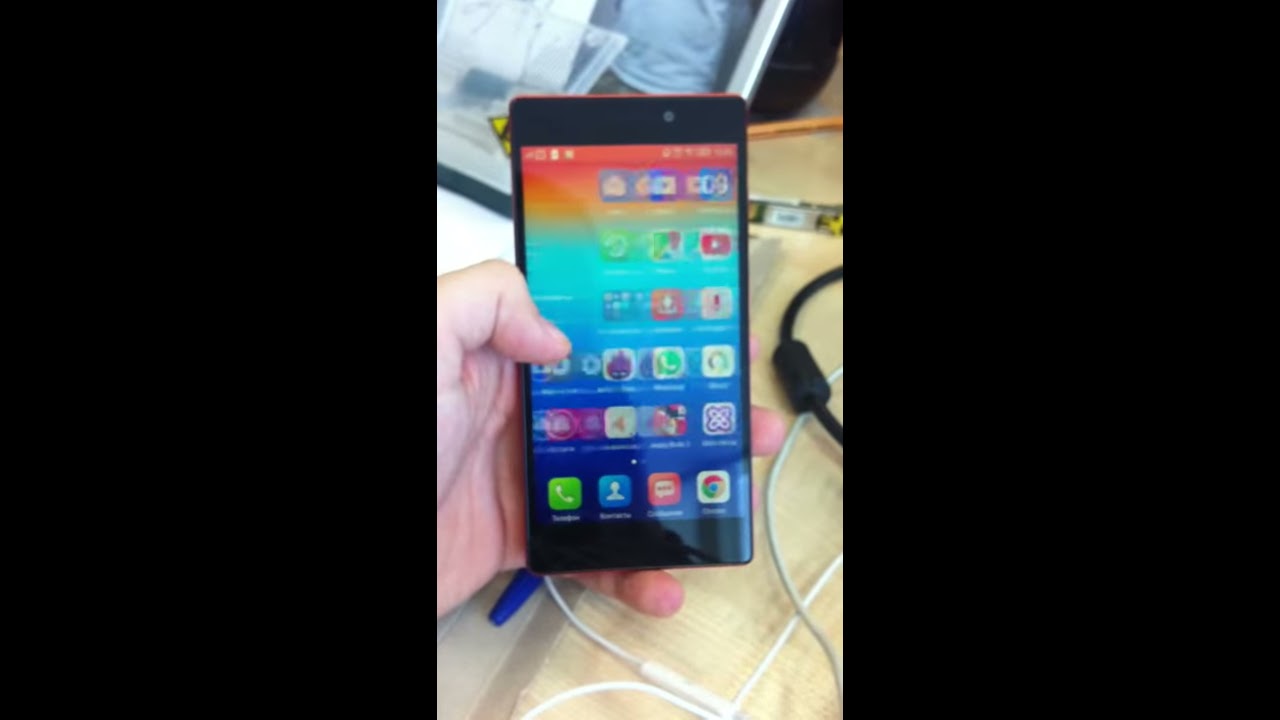The image captures a close-up of someone holding an Android smartphone in their left hand, with their thumb placed on the colorful screen. The phone's top and bottom are black, while the vivid screen displays a rainbow gradient background with shades of orange, red, turquoise, and blue, dotted with numerous app icons. The setting appears to be indoors, brightly lit, with a beige table as the backdrop. Scattered on the table are several black and white cable cords, weaving in and out, and some indistinct objects. The phone, centrally positioned along with the hand, stands out against the background clutter.